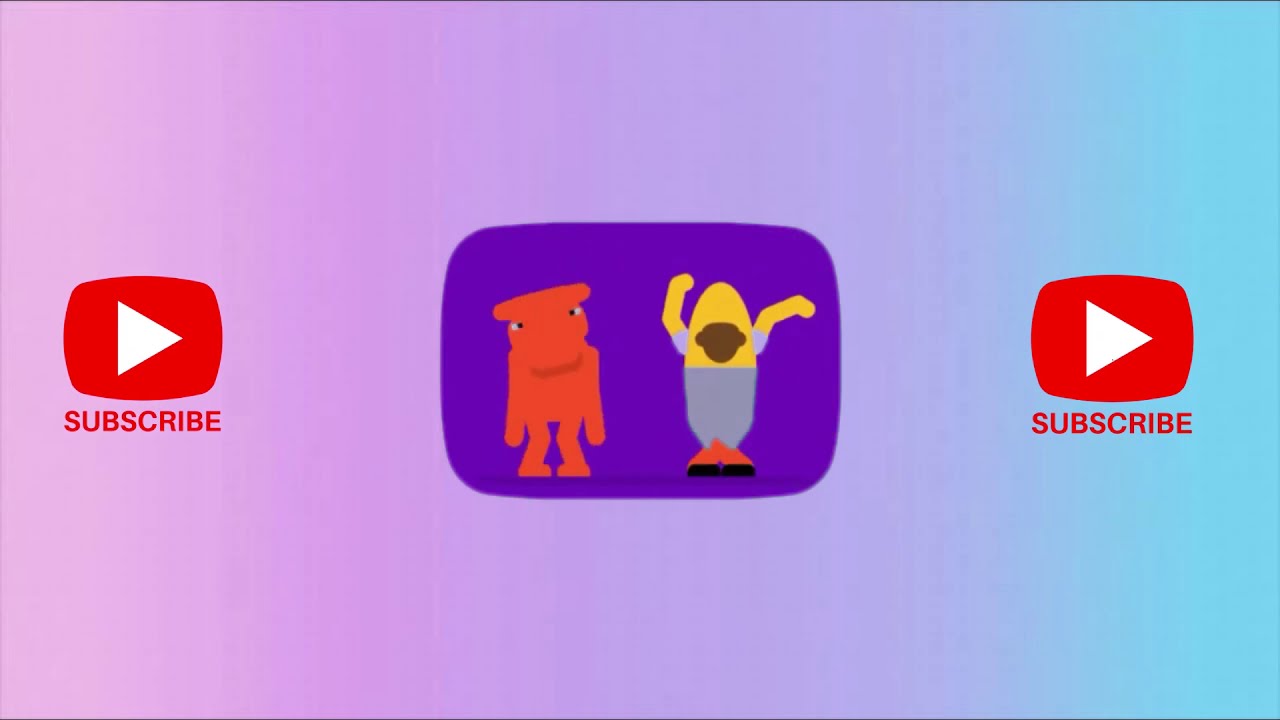This image appears to be an advertisement for social media, prominently featuring the YouTube play button logo. The background is a colorful gradient transitioning from pink on the left, through purple in the middle, to light blue on the right. On both the left and right sides of the screen, "SUBSCRIBE" is written in uppercase red letters, accompanied by the white triangle play button inside a red box with curved edges.

Centrally, there is a purple rectangle with rounded corners. Inside this rectangle are two characters. The character on the left resembles a short, stumpy, orange creature with a head that appears rat-like, possibly resembling a dinosaur or dragon. The character on the right looks like a yellow figurine, resembling a corn on the cob or a poorly drawn Minion, featuring a brown mouth, two arms, wearing grey pants or a skirt, and red feet. A large brown block protrudes from the middle of this character.

The overall design hints at a playful, eye-catching, and colorful advertisement aimed at enticing viewers to subscribe, leveraging familiar YouTube branding and whimsical character art to draw attention.